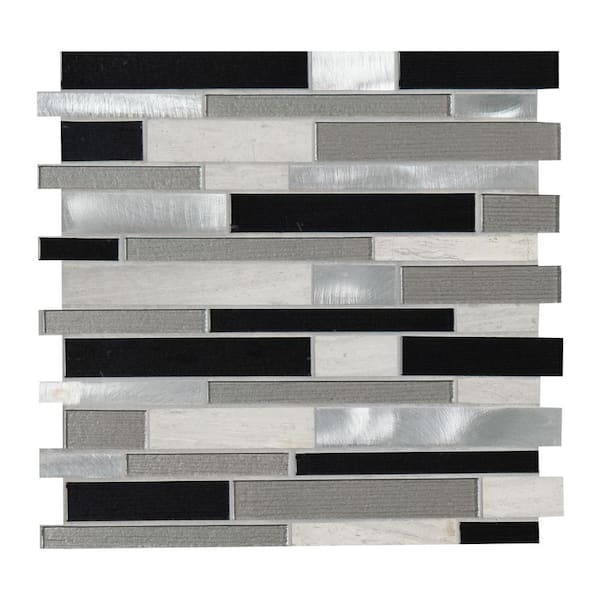This is a detailed square tile backsplash piece, often used in kitchen designs, featuring an intricate layout of long, thin, rectangular blocks. The tiles exhibit a variety of colors and textures, including solid black, translucent pearly white, metallic silver, gray, dark gray, and a stone-like gray. Each block seems to be set with a slight rhythmic imbalance, creating a visually balanced yet dynamic pattern. The texture of the blocks varies: blacks have solid textures, silvers are metallic, while grays are either wood-like or spackled. This realistic style of tiling, devoid of any identifying text or markings, rests against a plain white background. The meticulously alternating colors and textures of the blocks create an eye-catching yet harmonious design ideal for modern aesthetic settings.